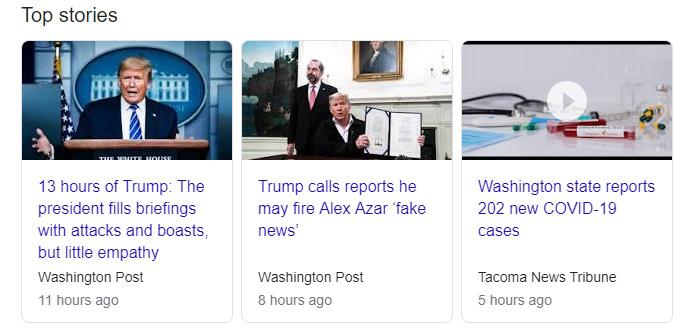The image depicts a media webpage showing the latest news stories. 

At the top left, under the heading "Top Stories," is a link featuring a photo of former President Donald Trump standing at a press conference podium at the White House. The link is accompanied by the headline: "13 hours of Trump. The President fills briefings with attacks and boasts, but little empathy." This story was published by the Washington Post 11 hours ago.

To the right of this, there is another story with a picture of two men in front of a portrait of George Washington. One man, dressed in a blazer and white collared shirt open at the top, is holding a large menu as if showing it to someone. The second man, wearing a black suit, white shirt, and pink necktie, stands behind him. The caption reads: "Trump calls reporters he may fire. Alex Azar, fake news." This article is also from the Washington Post and was published 8 hours ago.

The final image on the right appears to be from a video showing vials of blood and other medical items, suggesting a scientific or medical context. The caption states: "Washington State reports 202 new COVID-19 cases." This story was reported by the Tacoma News Tribune 5 hours ago.